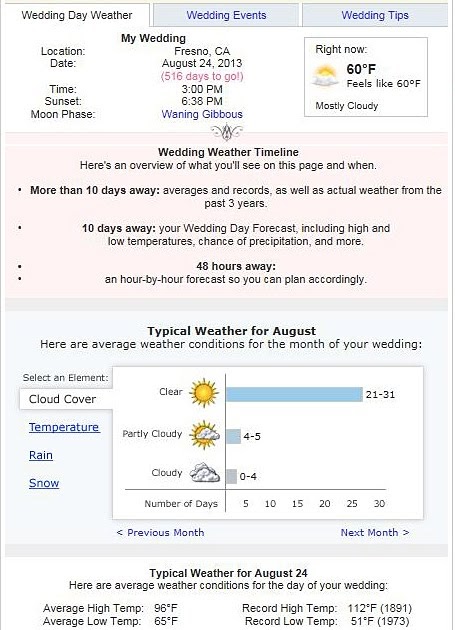This is a screenshot of a detailed wedding day weather report for Fresno, California, set for August 24th, 2013, exactly 516 days away from the current date. At 3 p.m., the temperature is 60°F and mostly cloudy, with the sun expected to set at 6:38 p.m. and the moon in its waning phase. The report features a "Wedding Day Weather Timeline," offering a comprehensive overview for planning purposes.

The interface includes clickable tabs for "Wedding Events" and "Wedding Tips" alongside the weather report. For dates more than 10 days in the future, it provides averages, records, and actual weather data from the past three years. Closer to the event, within 48 hours, it offers an hour-by-hour forecast.

Specifically for August 24th, historical data indicates typical weather with an average high of 96°F and a low of 65°F, while record temperatures have ranged from a high of 112°F to a low of 51°F. The report details expected elements like cloud cover, which is generally clear for this date. This comprehensive forecast allows for meticulous planning of wedding activities around anticipated weather conditions.